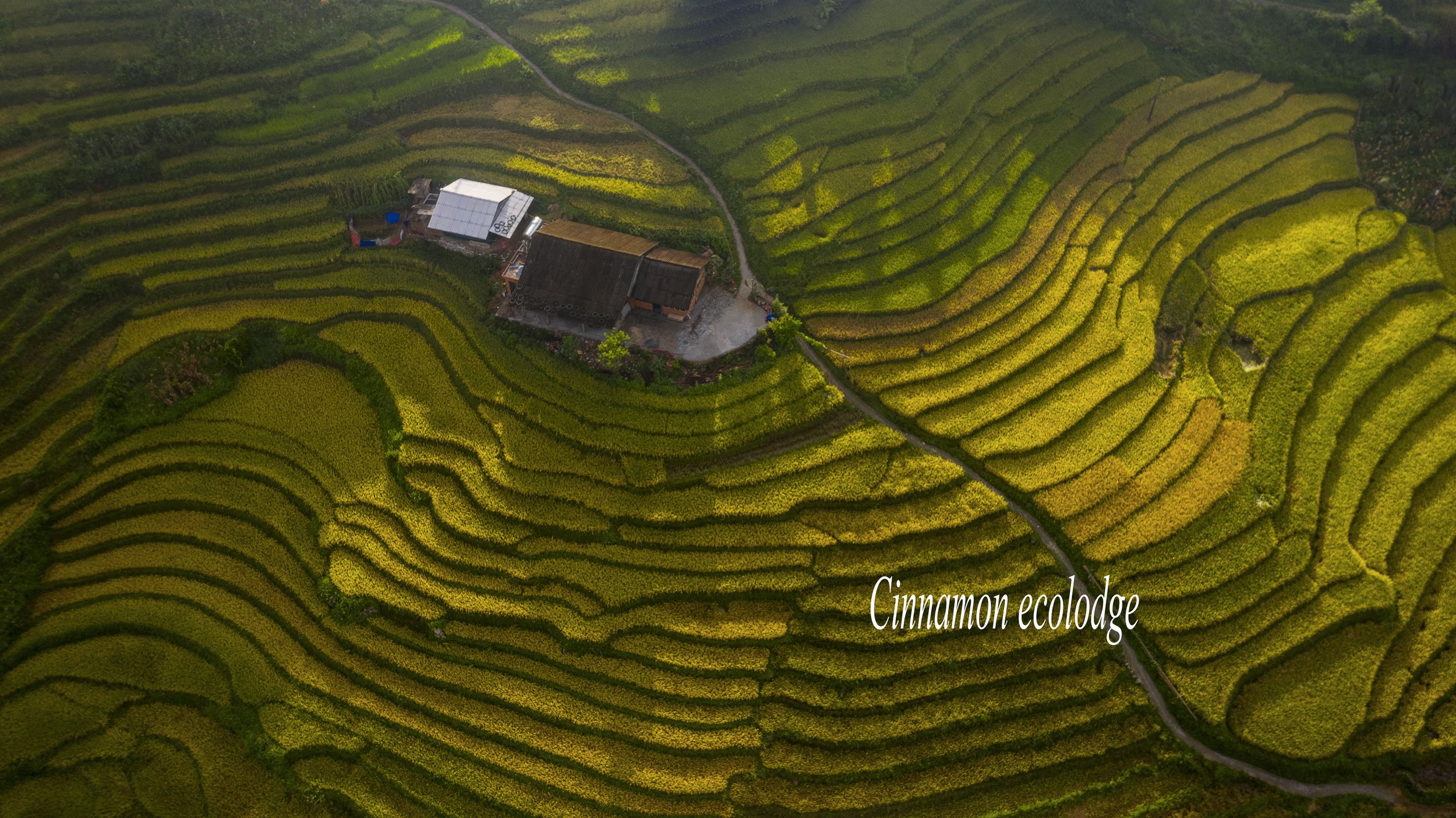This aerial photograph captures the expansive and intricate layout of the Cinnamon Eco Lodge nestled in what appears to be tiered agricultural fields, possibly tea or cinnamon. The terraced fields cascade down the mountainside in varying shades of green and yellow, creating a stunning patchwork that extends over a vast area. A roadway bisects the layered terraces, winding from the bottom right to the top right of the image. The center of the photograph highlights the lodge complex, which includes a farmhouse with a brown roof and an adjacent structure with a white roof, possibly a barn. Additional features include a parking lot and a few scattered trees around the lodge, casting long shadows suggestive of a setting sun. The overall scene exudes a sense of harmonious coexistence between the man-made and natural environments.